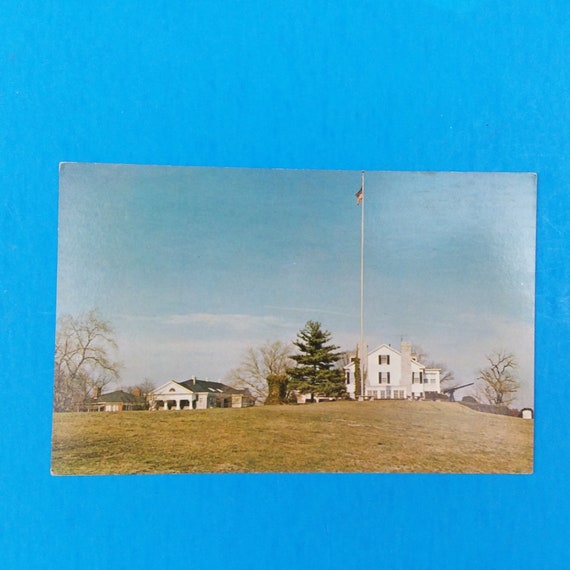This is an older photograph on a light blue background, featuring three buildings. In the center is a large, white, two-story residential house with a triangular roof and two gray chimneys. The upper floor has a single window facing front, while the ground floor features three windows. Attached to the house is a porch area with several tall windows. Directly in front of this house stands a tall flagpole flying an American flag in blue, red, and white. To the right of the flagpole is a tall, green, Christmas tree-like pine tree, with another tree to its right that appears to be either dead or bare, indicating early in the year with sparse leaves. To the far left of the image are two smaller commercial buildings, one with a gray roof and the other with large white pillars in the front. The background sky is blue with some scattered white clouds, and the ground at the bottom of the image is a mix of green and brown grass. The edges of the photograph are frayed, suggesting its age.